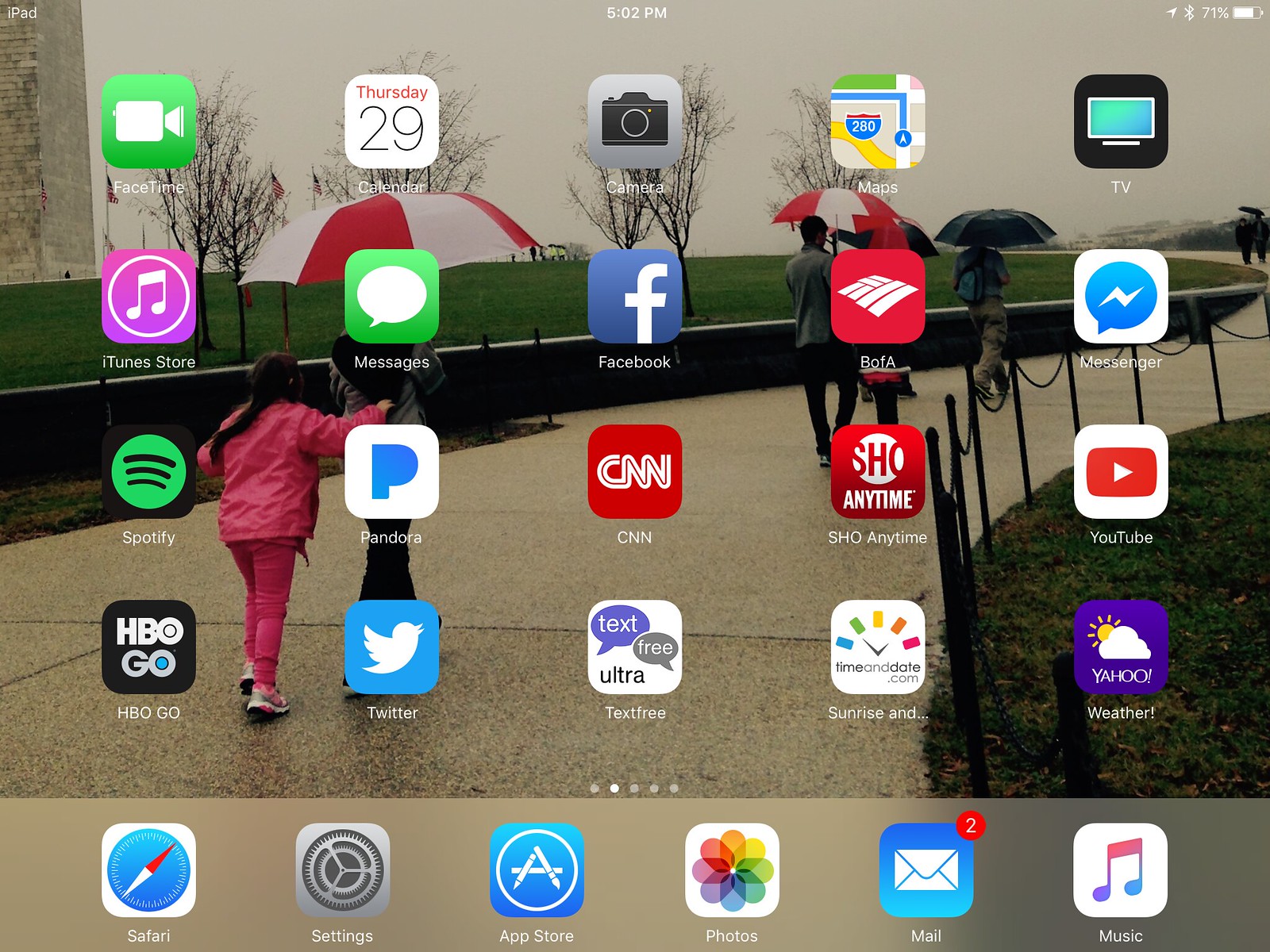The image showcases the screen of an iPad, which is identifiable by the small text "iPad" in the upper left corner. Additionally, the screen displays standard status icons including the time and battery level at the top.

The iPad's background wallpaper features a vivid and bustling scene depicting several people walking along a sidewalk with umbrellas, possibly in a rain-soaked urban setting. Overlaying this backdrop are numerous app icons neatly arranged in a grid.

Among the visible apps on the screen are:
- FaceTime
- Messages
- Calendar
- Camera
- Maps
- TV 
- Messenger
- Bank of America
- Facebook
- iTunes Store
- Spotify
- Pandora
- CNN
- Showtime Anytime
- YouTube
- Yahoo
- Textfree (a messaging app)
- Twitter
- HBO GO

At the bottom of the screen, in the dock, are additional frequently-used apps:
- Safari
- Settings
- App Store
- Photos
- Mail
- Music 

Each icon is clearly displayed, contributing to a highly detailed and organized interface on this iPad screen.